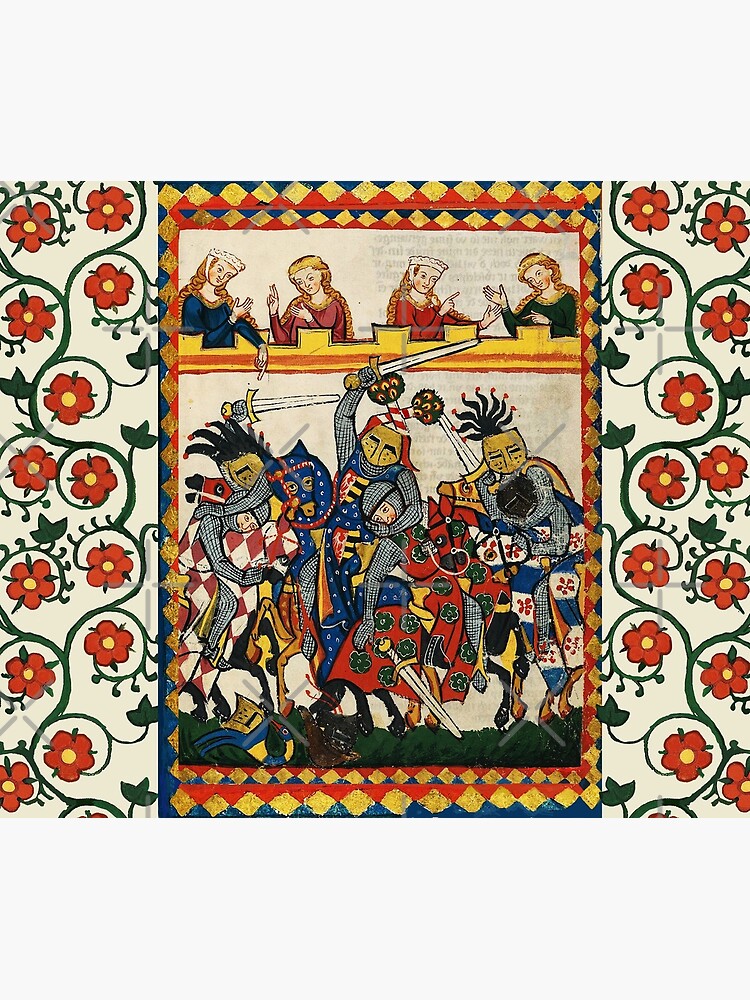This is a medieval-style painting, featuring an ornate and detailed battle scene set within the confines of a decorated border. The painting likely mimics pre-Renaissance artistry and creates a highly stylized depiction of knights engaged in combat, not necessarily fighting to the death, but perhaps partaking in a sport-like joust within an arena. The arena is bordered by a wall on top of which sit noble ladies, adorned in vibrant attire—plum, blue, red, and green—watching the skirmish below. 

The painting is framed with dual borders, the inner one adorned with intertwining vines and small red flowers with yellow centers on a white background, and the outer border featuring an intricate pattern of red, blue, and golden diamonds. In the center of the image, knights in colorful garb, possibly on stylized horses, wield swords aloft, seemingly locked in intense combat. The vivid colors and meticulous detail of the figures and scenery convey a sense of grandeur and complexity typical of medieval artistic traditions.